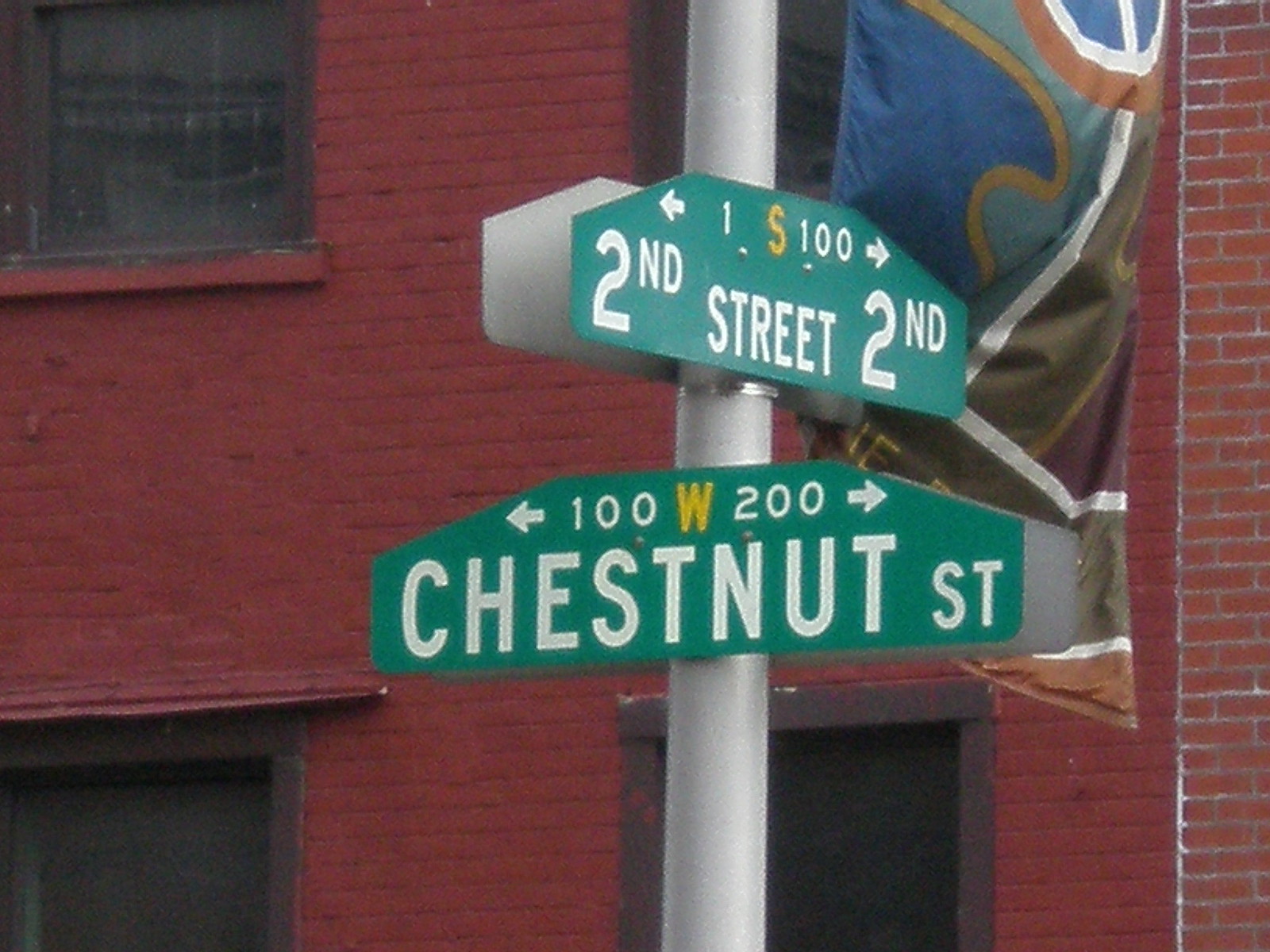The photograph captures a street sign mounted on a grey metal pole. The background showcases a red brick building, likely an apartment complex, with several visible windows. One window, located in the top-left corner, features a brown frame and a large vertical rectangular pane. Another window is visible at the bottom left, and behind the pole, a portion of a third window can be seen, with an additional window rising from the bottom of the image. 

A flag with irregular patterns and various colors, including blue, green, brown, dark yellow, and white, hangs down in the scene. 

The street sign features two panels: the top panel is green with white and yellow text. It has a left-pointing white arrow followed by the text "1 S 100," and a right-pointing white arrow with "Second Street" written beneath it. 

The second sign, attached below the first, points slightly to the left and includes a similar arrangement of arrows. This sign has a yellow "W" flanked by the numbers "100" to the left and "200" to the right. Below this, in white capital letters, it reads "Chestnut St."